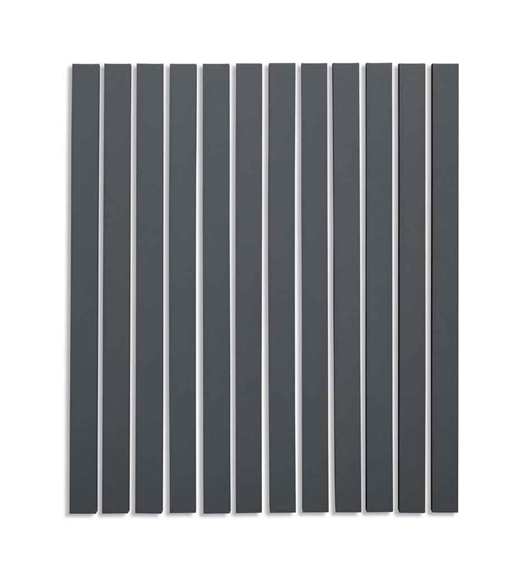The image features a simple, vertically oriented, rectangular graphic with a white background and a series of dark gray vertical lines. There are 12 dark gray lines uniformly spaced across the image, creating columns that resemble curtain blinds or elongated rectangles. Each gray line is separated by narrow white spaces that are approximately one-fifth the width of the gray lines themselves. The gray lines appear to have a slight 3D effect, with subtle shadows on their left sides, adding a touch of depth to the otherwise minimalist design. The image contains no text or additional colors, emphasizing its stark, monochromatic aesthetic.